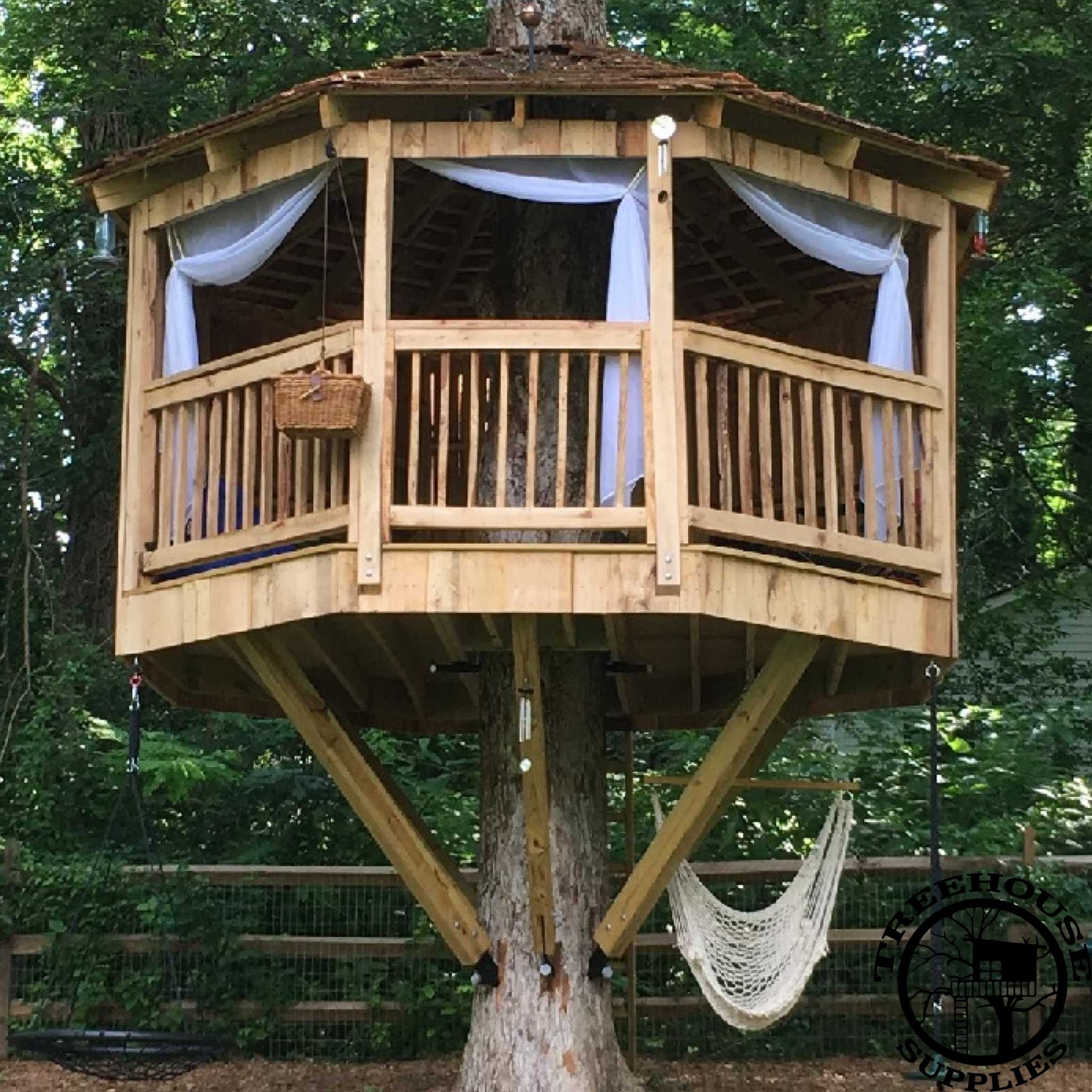This is a high-quality color photograph of a large, elaborate treehouse, prominently featuring a logo in the bottom right corner that reads "Treehouse Supplies" in black, accompanied by a circular design of a treehouse. The treehouse itself is octagonal, supported by a sturdy, wide trunk that passes through its center. The structure is equipped with three visible railings and square open areas, giving it a hut-like appearance. White curtains hang in the openings, adding to its aesthetic. Inside the treehouse, there is a basket pulley lever system, a wind chime, and a bird feeder, adding functional charm. Below, a white leather hammock is suspended, providing a relaxing spot for lounging. A wooden fence with wires runs along the back, and lush green leaves from surrounding trees frame the background, completing the scenic and serene setting. There are no individuals in the image, allowing full focus on the captivating treehouse and its details.